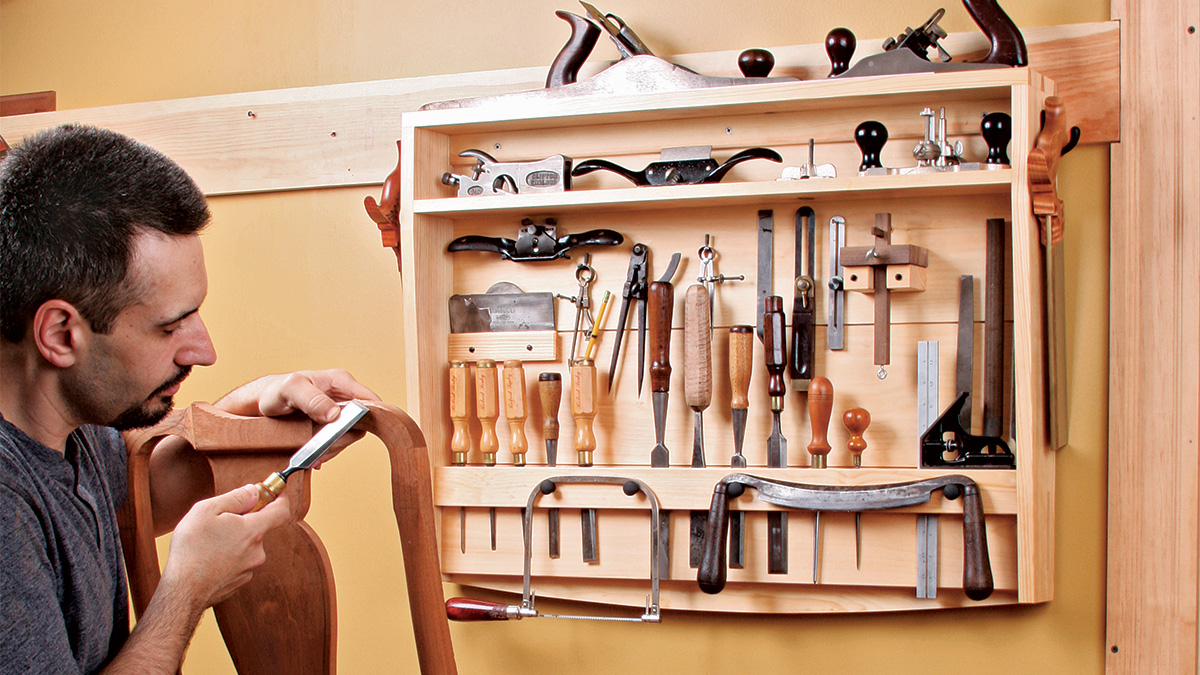In this detailed photograph, a man is engrossed in woodworking within his shop. Positioned to the left, he is captured from his right side, revealing his black hair and a short black mustache and beard. He wears a gray shirt and is meticulously using a small carving tool to shape the upper back of what appears to be a walnut chair. His right hand holds the chisel part against the wood while the handle is gripped in his other hand. The workspace around him is an organized array of various woodworking tools. Directly in the background, a wooden cabinet is filled with tools, many of which have light brown handles and metal chisel blades. Above and around the cabinet, more tools are visible, including sanders with black handles, saws, files, clamps, and different picks. Additionally, the tools are attached to shelves fastened to a yellow wall, supported by a horizontal board running the length of the wall, with nails, screws, and fasteners indicating the potential for more storage or support for additional shelves.